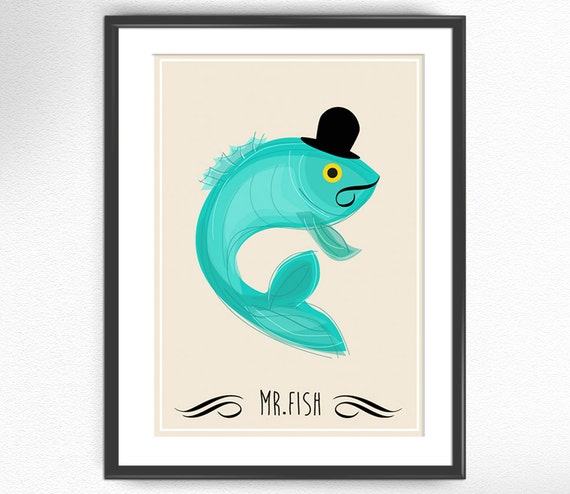The image depicts a whimsical and cartoonish teal fish with a curling body. The fish wears a small, rounded black top hat and sports a curly black mustache. Its eye is drawn in yellow with a black center. The fish's fins and tail, also in shades of teal, are detailed and distinct. The background of the artwork is a creamy off-white color. The image is framed in a black frame with white matting, giving it a finished and professional appearance. Below the fish, centered in black lettering, it reads "Mr. Fish," flanked by decorative black squiggly flourishes on either side. The entire picture is mounted on a white wall, emphasizing the playful and charming nature of the framed print.